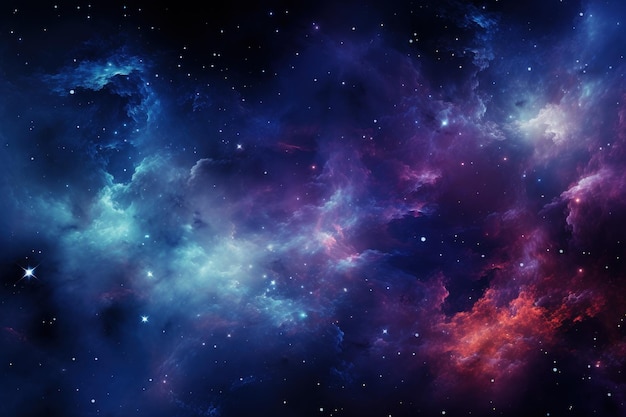This nighttime image captures a stunning view of a galaxy set against a pitch-black sky. The photograph, taken outdoors, is dotted with hundreds of stars of varying sizes and brightness, creating a celestial spectacle. A vibrant nebula spans from the left to right, dominating the center of the frame and adding a puffy, cloud-like texture. The nebula's vivid colors range from dark and light blues to purples, reds, pinks, and even coral, creating a dynamic and striking visual impact. At the bottom right, intense shades of orange and purple mingle, while the upper left is predominantly blue with subtle hints of purple. The upper right section, although smaller, continues the interplay of lighter colors. The stars, some sparkling brightly and others appearing like distant white specks, are nestled amidst the swirling gases, which gives the nebula its stunning coloration and shape. The overall effect is reminiscent of an explosion or a chemical reaction in space, evoking a dramatic, almost surreal atmosphere.